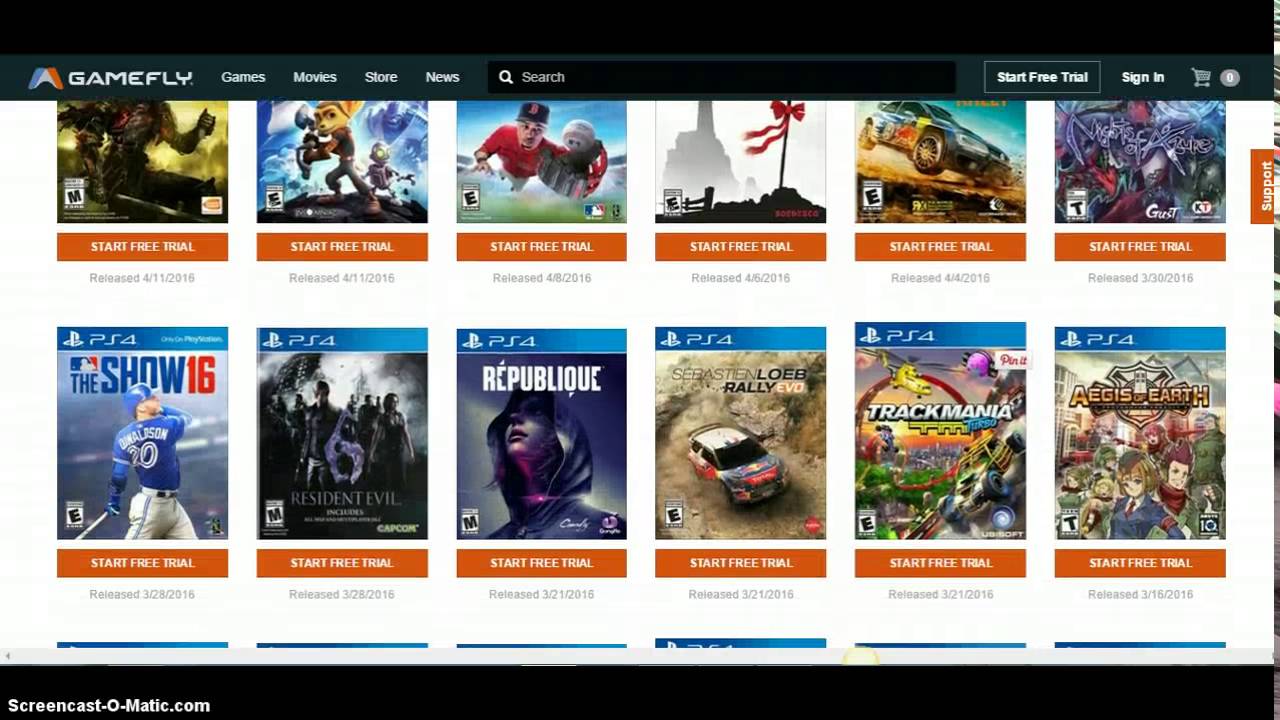This is a detailed and cleaned-up caption of the provided image description:

---

The image is a horizontal rectangular screenshot from the GameFly website, prominently displaying a collection of PlayStation 4 (PS4) game covers. The layout features noticeable black headers and footers at the top and bottom, occupying approximately 10% of the image's height. The rest of the image consists chiefly of colorful game covers arranged against a white background.

At the top, the black header contains the GameFly logo and navigation options. The GameFly logo is on the left, depicted as a video game controller with an orange right handle and a blue left handle. Adjacent to the logo, the text "GAMEFLY" appears in all capital letters. To the right, four clickable options: "Games," "Movies," "Store," and "News," are presented in white text. Below the navigation, a search bar spans across the header, featuring a magnifying glass icon, the word "Search" in white, and an interactive "Start Free Trial" button followed by a "Sign In" link in bold white, and a shopping cart icon. There is also a gray circle icon whose details are indistinguishable.

The central portion of the image showcases 12 PS4 games in two rows of six, with the top row slightly cut off. Each game cover, in portrait orientation, features a detailed and colorful design. The top border of each cover shows a medium blue strip with "PS4" and the PlayStation logo in white.

Here are the game covers in the visible second row, from left to right:

1. **The Show 16**: A baseball-themed cover featuring Josh Donaldson of the Blue Jays in a blue shirt and helmet, white pants, mid-swing with a bat. The title "THE SHOW" is in white, with "16" in red.
2. **Resident Evil**: Depicts zombie-like figures wandering, signaling its survival horror theme.
3. **Republique**: Highlights the head and shoulders of a woman gazing upwards, wearing a hood, conveying a sense of mystery.
4. **Sebastien Loeb Rally Evo**: Displays a rally car speeding on a dirt road, emphasizing its racing theme.
5. **TrackMania**: A vibrant, chaotic cover with cartoonish colors and elements indicative of high-speed racing and stunts.
6. **Aegis Earth**: Anime-style artwork featuring a group of characters standing together, suggesting a narrative or RPG theme.

Each game cover in the second row is topped and tagged with a release date, such as "Released: 3/28/2016" for "The Show 16".

The top row is partially visible, showing only the bottom portions of the game covers:
- The first cover appears to display a character holding a sword.
- Subsequent covers partially show elements, like a multicolored racing car in the fifth slot.

At the very bottom, the black footer includes the text "Screencast-O-Matic.com" in white in the lower-left corner, potentially indicating the screen capture source.

---

This caption paints a comprehensive visual description, providing details for each section of the image.